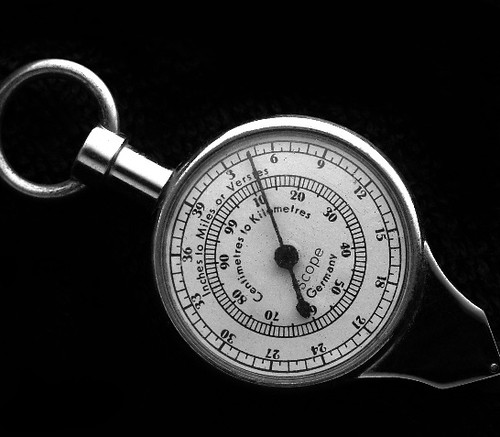The image features an intricate gadget, prominently displaying a meter angled diagonally. At its center lies a black dial positioned between the numbers 3 and 6. Encircling this central dial, numerals range from 3 to 39 in increments of three: 3, 6, 9, 12, 15, 18, 21, 24, 27, 30, 33, 36, and back to 39. Alongside the numbers, there are labels indicating measurements in inches, miles, or verses.

Encircling this innermost ring is another ring starting with the number 99, which progresses incrementally by tens up to 90: 10, 20, 30, 40, 50, 60, 70, 80, and then 90. Measurements in centimeters to kilometers are also marked within this ring. Near the base of the gadget, the text "Scope Germany" is clearly visible, denoting its origin.

In the background, the gadget is set against a white backdrop with all characters and markings in black, including the central dial. On the right-hand side of the image, there's a pyramid-shaped structure forming part of the handle. At the top left, there's a small gray cylindrical base attached to a silver ring, which stands out against a contrasting black background.